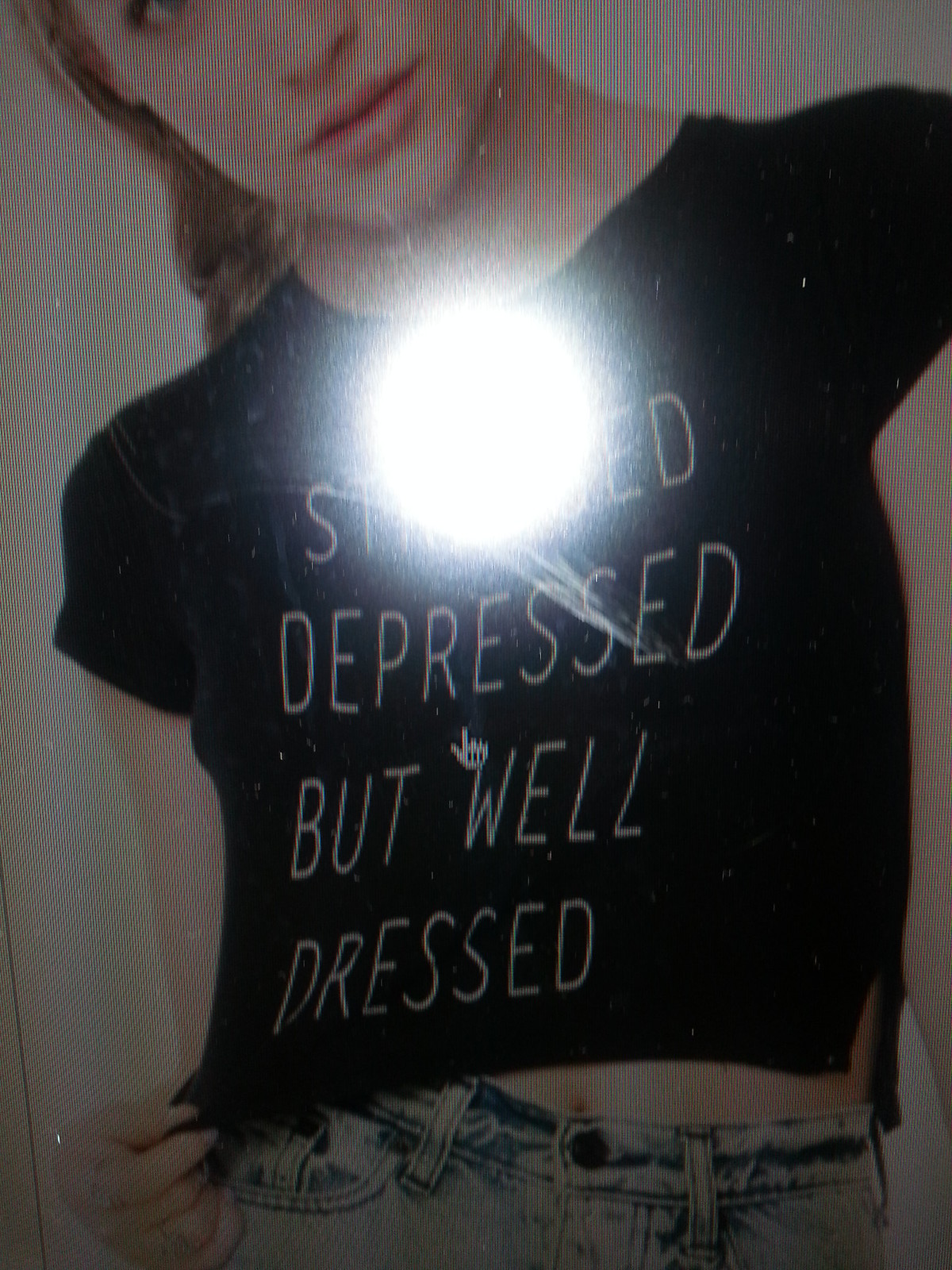This digitized image captures a young, blonde-haired, Caucasian woman with long light brown hair, wearing a black, short t-shirt that reveals part of her midriff and features the white text "stressed, depressed, but well-dressed." The t-shirt also has a v-shaped cut on the side, and she pairs it with blue skinny jeans. The woman's face is slightly cropped out, but her pink lipstick is visible. The image has a bright white flash or glare at the center, indicating it is a photo of a computer screen displaying another photo, resulting in a blurry and distorted quality with a riveted or lined filter effect. The background is beige, and a mouse cursor hovers near the picture, suggesting it is about to click on it.